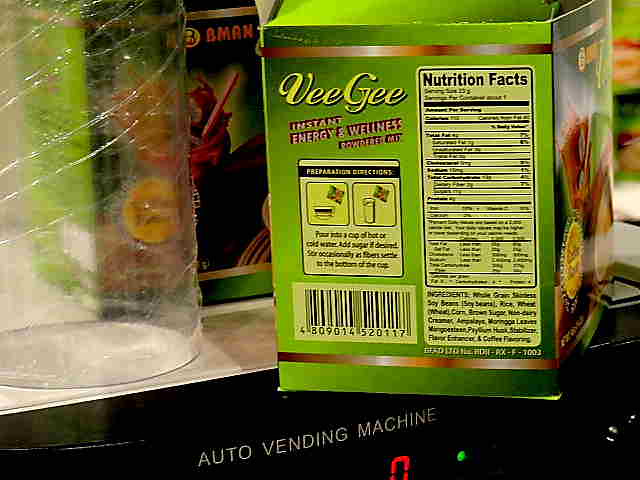The image depicts a product known as VG's Instant Energy and Wellness Powdered Mix, packaged in a large green square box prominently displayed at the center. The box features detailed instructions on the side, suggesting that the mix can be prepared by pouring it into a bowl or a glass, indicating its primary use as a drink mix. The setting appears to be atop an "Auto Vending Machine," evidenced by visible text below the product. Surrounding the main box are additional boxes of the same product, alongside what appears to be a plastic or glass cup, suggesting a demonstration or a promotional setup. The product's nutritional facts are also visible, adding to its detailed presentation.